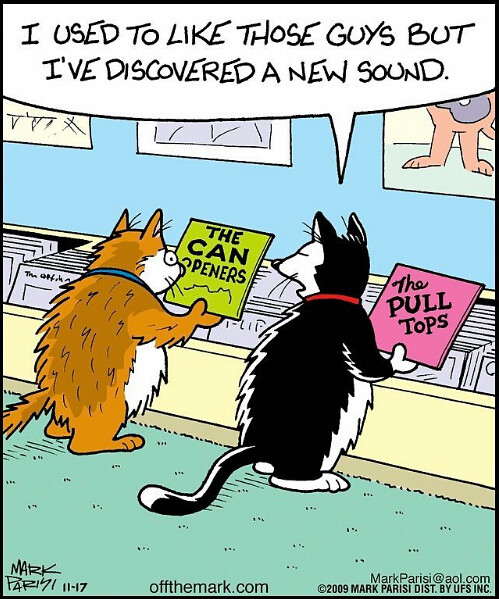This comic strip or postcard depicts two anthropomorphized cats in a vintage-style record store. Set against a blue wall adorned with partially visible pictures, the scene features the cats standing on a green carpet amid yellow record bins filled with grey records. On the left, an orange-and-white cat with a blue collar holds a green album labeled "The Can Openers." To the right, a black-and-white cat with a red collar holds a pink record titled "The Pull Tops." A word bubble above the black-and-white cat reads, "I used to like those guys, but I've discovered a new sound," humorously alluding to cats' reaction to can openers. The comic is signed by Mark Parisi, with credits and contact information dispersed across the bottom: “Mark Paris, 11-17,” “OffTheMark.com,” and “Mark Parisi, at AOL.com,” alongside the copyright notice, “2009, Mark Parisi, DIST, by UFS, Inc.”